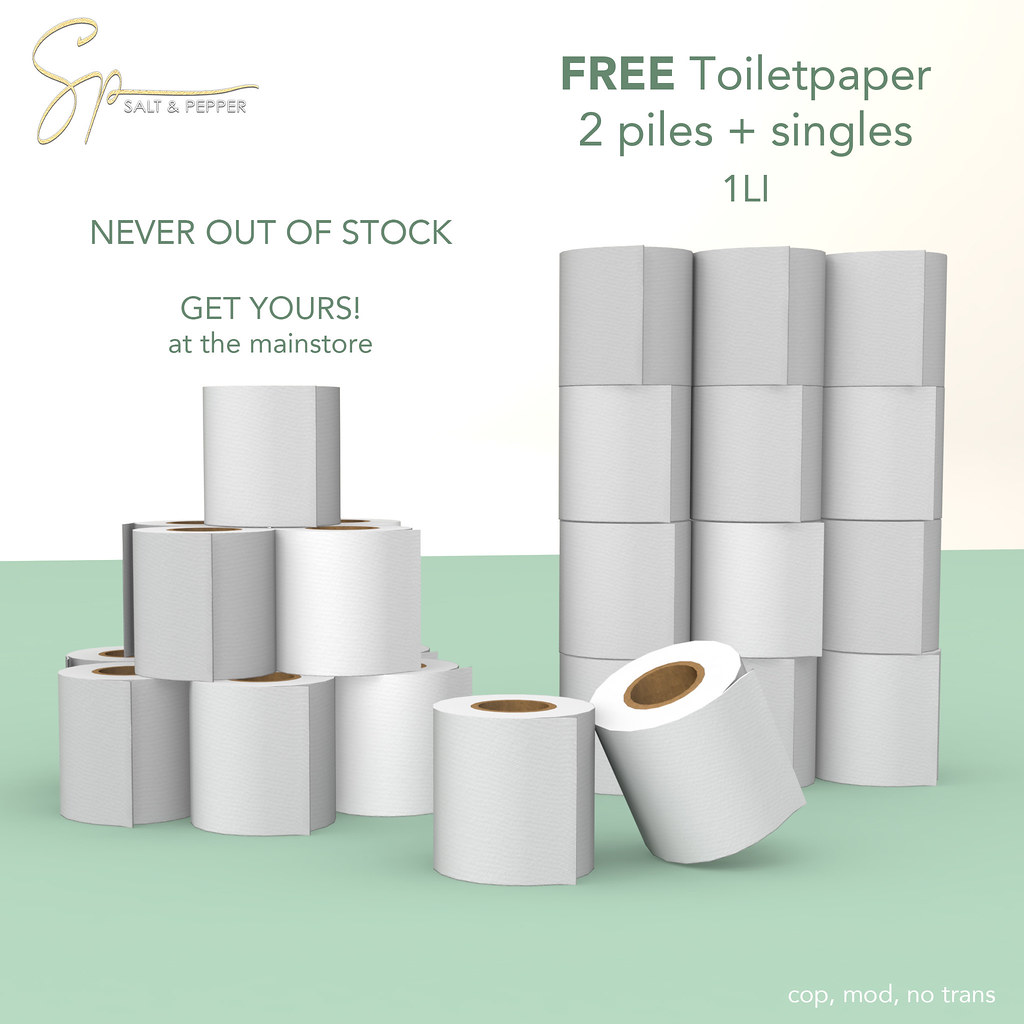This is a square format color illustration featuring two distinct stacks of toilet paper rolls positioned against a bicolor background—mint green on the bottom and cream on the top. The stack on the left forms a pyramid, arranged in a 3-2-1 configuration from bottom to top, while the stack on the right consists of four rows, each containing three rolls. In the foreground, two lone rolls are placed, one of which touches the other diagonally. 

Dominating the top left corner is a gold logo with the cursive initials "SP," followed by the words "salt and pepper" in small letters. Adjacent to the logo, in bold green text, are the words "FREE TOILET PAPER," with the term "FREE" in all caps. Beneath this, the text continues in dark green stating, "two piles plus singles one LI." 

Over the pyramid stack on the left, white text in all capitals reads, "NEVER OUT OF STOCK!" followed by "Get yours at the main store" in lowercase. The very bottom right of the image features white text that reads, "cap, mod, no trans." The illustration combines graphic design elements and typography to arrange the image thoughtfully and coherently.